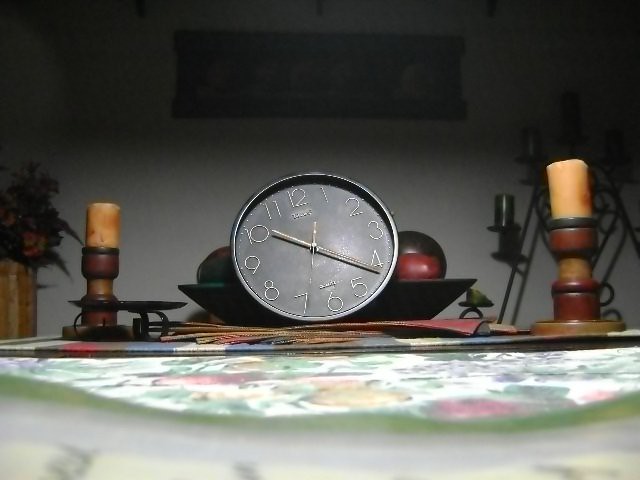The image features a round analog clock prominently displayed on a table, with its hands indicating approximately 10:22. Behind the clock rests a bowl containing several apples, contributing a touch of vibrancy and color to the scene. The table, which appears to be either a kitchen or dining room table, is adorned with a flowery tablecloth, adding a homely and decorative element to the setting.

Flanking the clock and the fruit bowl are two chunky wooden candlesticks, each holding a partially burnt cream-colored candle, suggesting recent use or a warm, lived-in atmosphere. In the background, attached to a white wall, there is a long, rectangular object that is slightly ambiguous—it might be a picture frame, a shelf, or perhaps a small, narrow window, its precise identity obscured but it adds a vertical element to the composition. Overall, the arrangement creates a cozy and inviting scene, rich with everyday domestic details.